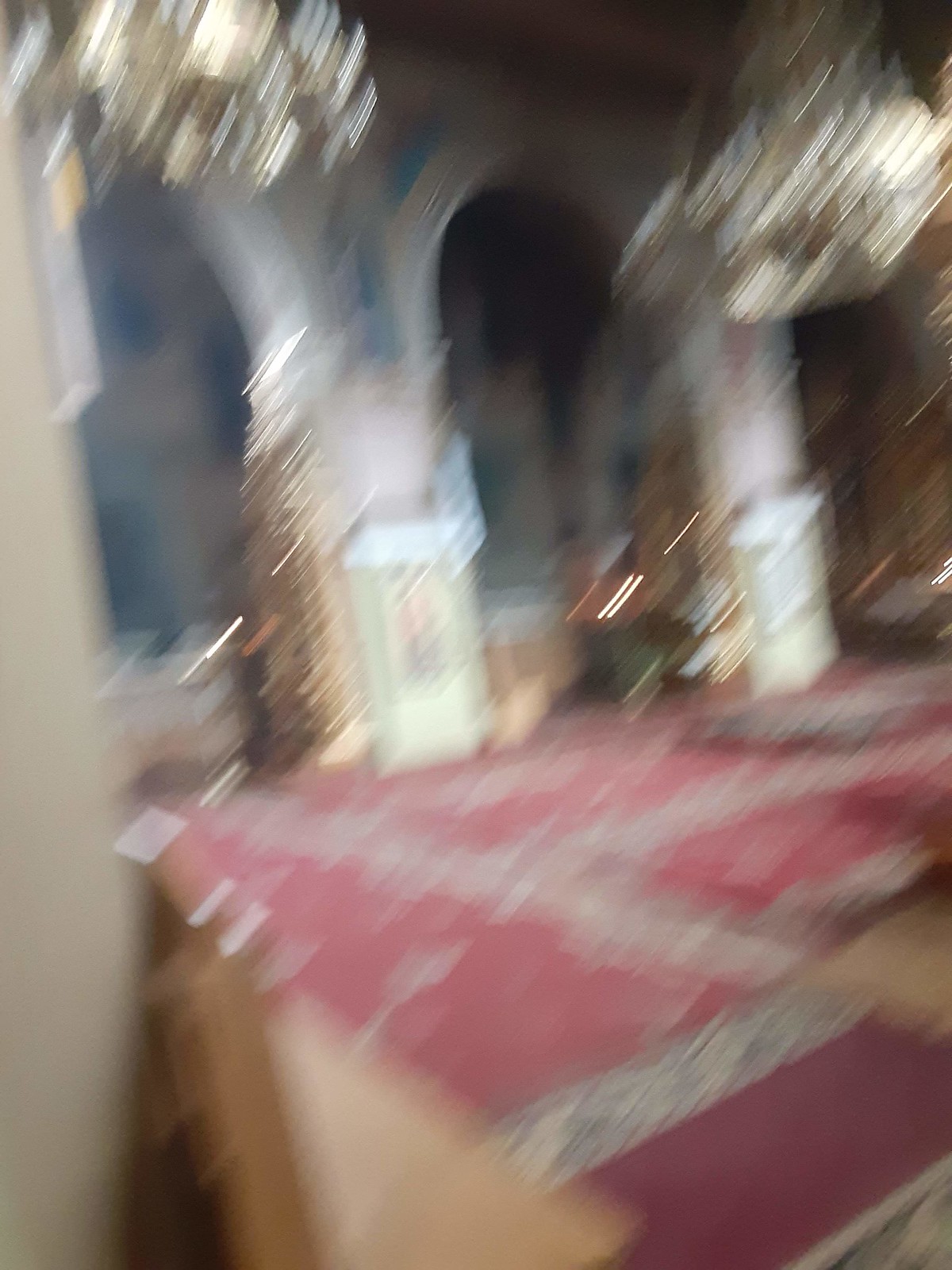In this extremely blurry image, there appears to be a couple of structural objects positioned on a tablecloth. At the bottom of the image, a dark brown, vertically oriented shape is visible, possibly part of the structures. To its right, a tan, rectangular object can be seen from two sides, suggesting a three-dimensional form. The tablecloth beneath these objects is dark red with a design featuring gray stripes.

Above the table, the structure begins to take shape, highlighted by a white square in the center, reminiscent of a pillar that might support a building. Another similar structure is visible to the right. At the top of the image, two indistinct chandeliers can be seen, characterized by gold and gray tones, further adding to the architectural elements within the scene. Despite the lack of clarity, the objects suggest an intricate setting with both structural and decorative components.